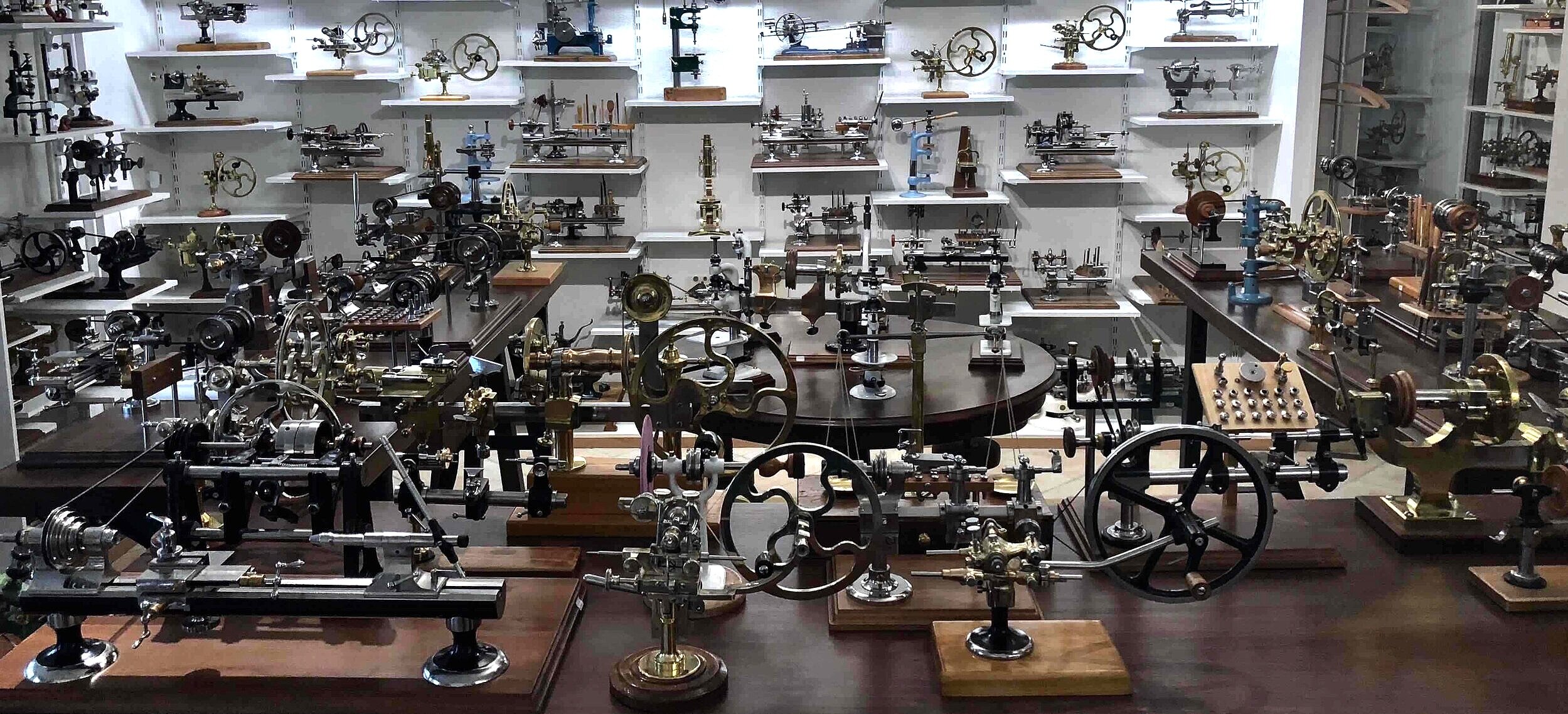The photograph depicts a detailed display inside a museum, showcasing an extensive collection of vintage sewing machines. The room is filled with multiple brown tables, both rectangular and round, and white floating shelves mounted on the walls. Each surface is laden with various models of sewing machines, characterized by distinctive mechanical designs featuring wheels, attachments, and cranks. These intricate machines include both hand-cranked and early motorized versions, reflecting different eras and styles. One notable machine, located on the bottom right, is set on a rectangular brown platform with a needle on one side and a large crank handle on the other. The arrangement of these historical artifacts on desks and shelves creates an organized yet densely packed display, emphasizing the ingenuity and evolution of sewing technology over time.